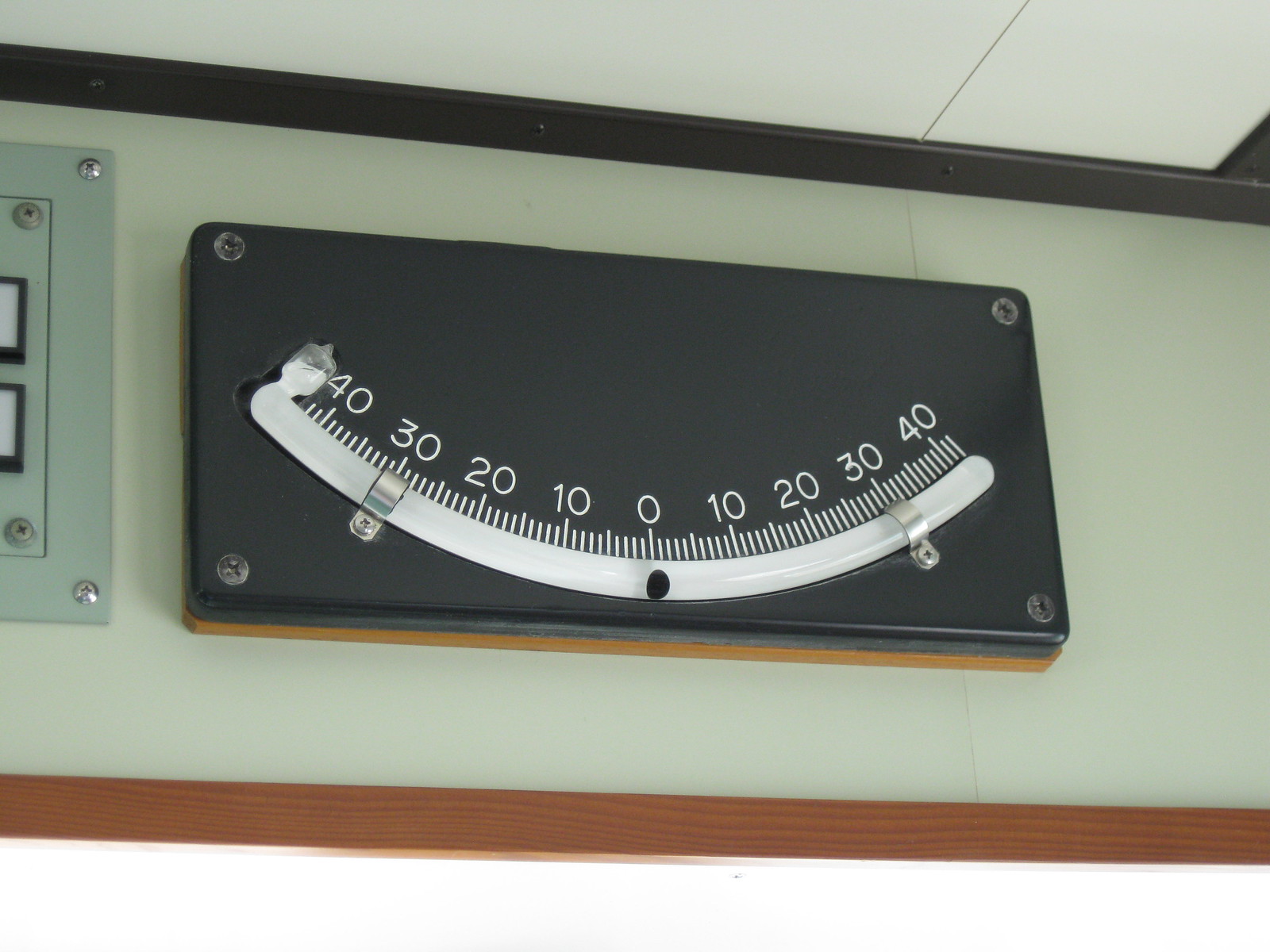This image features an unconventional, curved measurement device resembling a thermometer but styled more like a segmented light tube. The device starts at a central point marked zero and curves to the right with increments labeled 10, 20, 30, and 40, each segment delineated with smaller intervals. A larger line marks the midway points, suggestive of 5, 15, 25, and 35, which gives the impression of measuring units roughly analogous to inches. This same pattern continues symmetrically to the left, extending outward in equal increments.

The overall structure creates a curvature reminiscent of a smile, accentuated by a soft, glowing light that emanates evenly along the segmented scale. This entire apparatus is mounted on a black plaque, securely bolted to a wall, and is flanked by an adjacent panel suggesting the presence of additional measurement or information tools. The angle of the photograph reveals part of the ceiling, hinting that the installation is positioned relatively high on the wall.